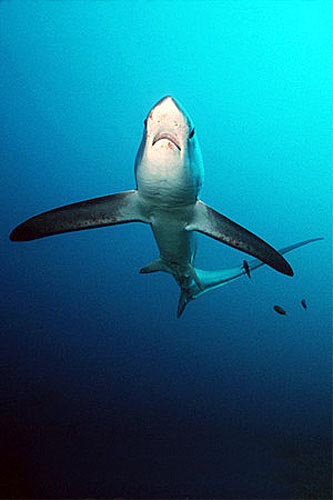This underwater photograph captures a dramatic scene of a shark swimming in the ocean. The photographer has taken the shot from beneath and slightly in front of the shark, resulting in a striking view of the shark's head pointing upward, with its fins outstretched toward the center of the image. The shark's underside is white, while its sides are a mix of gray and teal, and its fins have dark edges. The water transitions from an almost black at the bottom to a light sky blue at the top, highlighting the sunlight filtering through the shallower water. The shark's black eyes and open mouth add to its menacing presence. Surrounding the shark, specifically near its long, pointy tail, are several small black fish. The overall composition, with the gradient of the water and the positioning of the shark, evokes a cinematic quality reminiscent of a movie poster like "Jaws."